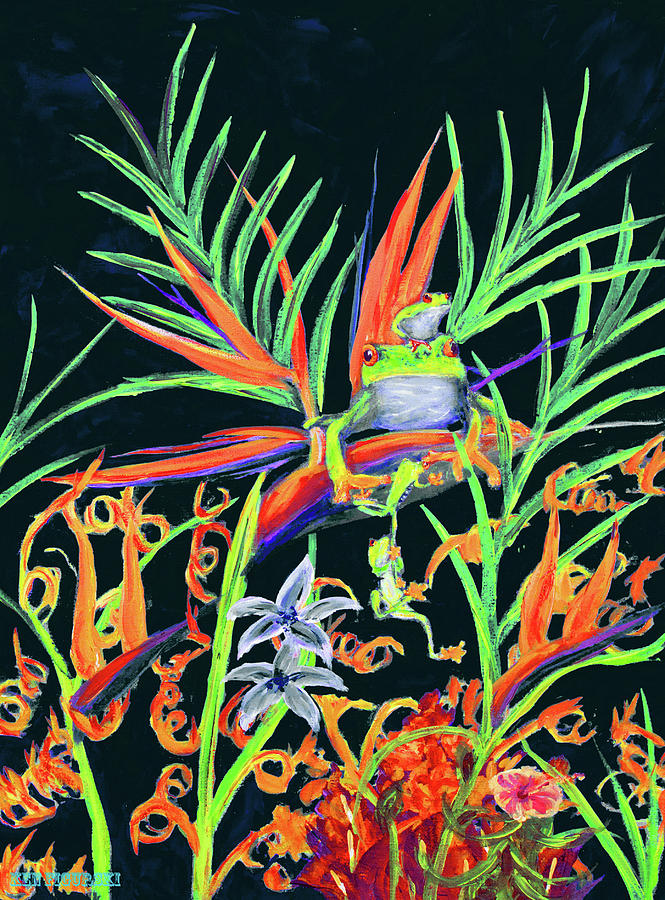This vibrant painting, set against a stark black background, depicts a richly detailed tropical jungle scene. Predominantly, it features lush green vegetation adorned with splashes of tropical colors such as orange, red, and hues of purple-blue. Among the dense foliage and vibrant flowers, a striking scene unfolds: a large green frog with a white underbelly and orange legs clings to a plant, seemingly defying gravity. Perched on its head is a smaller frog, adding a whimsical touch, while another frog dangles below, creating a lively trio centralized to the right of the composition. The plants, including ferns and vines, extend from a thick, colorful base, gradually tapering off towards the top where the black background dominates. Intricate flowers of blue and pink add further detail. The painting also features text in blue at the lower left corner, presumably the artist's name, although it is partially obscured by the vibrant orange and green foliage.